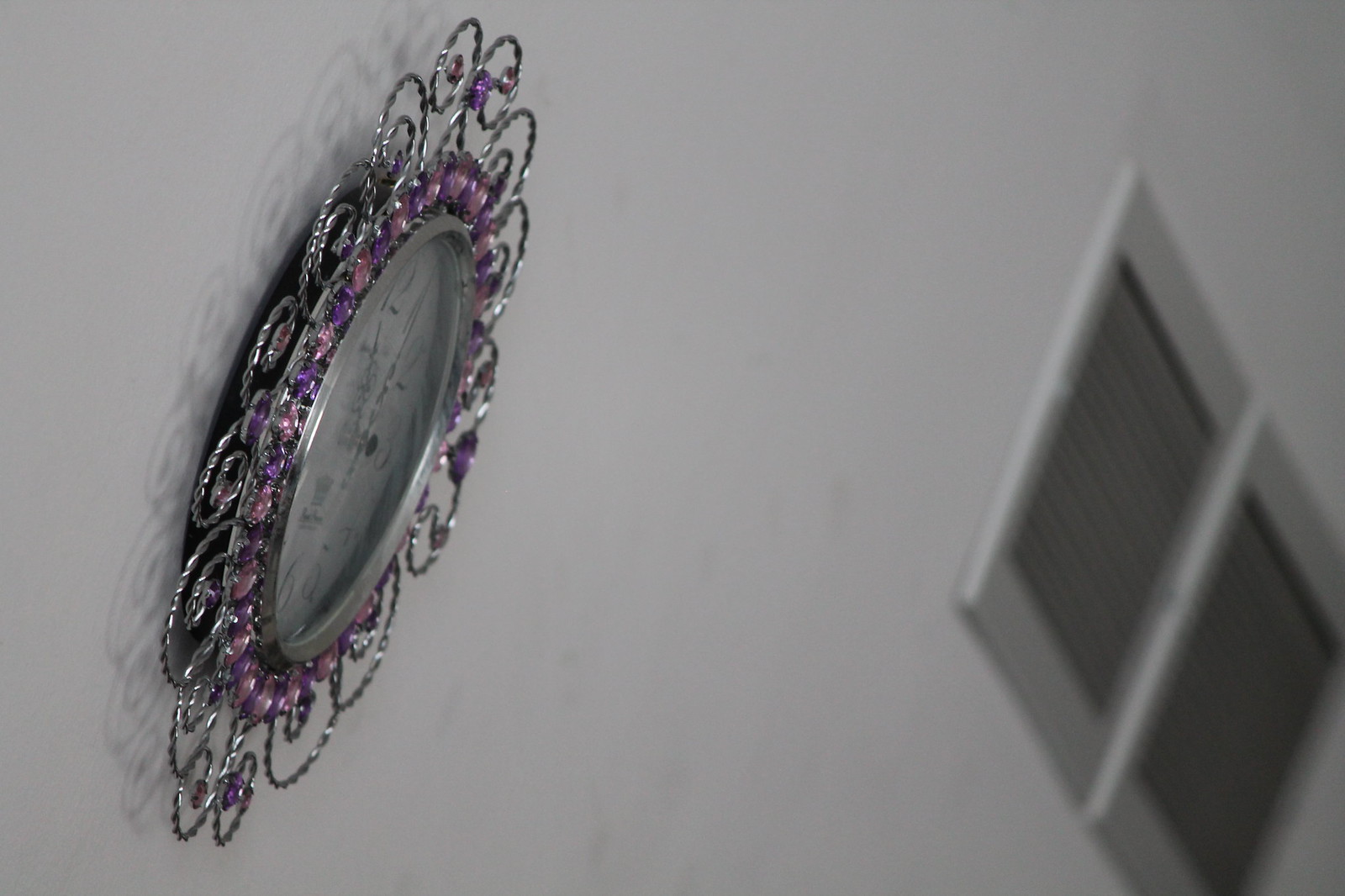The image captures a minimalist, white wall. On the right-hand side, a rectangular air vent with gray slats and a central dividing line is clearly visible. The focal point of the picture, however, is positioned to the left—a wall clock captured from a side angle. The clock's face is white and encircled by intricate detailing, including purple beading and metallic twine arranged in a zigzag pattern. This elegant combination of silver and beading accents highlights the face of the clock, making it stand out against the simplicity of the wall.